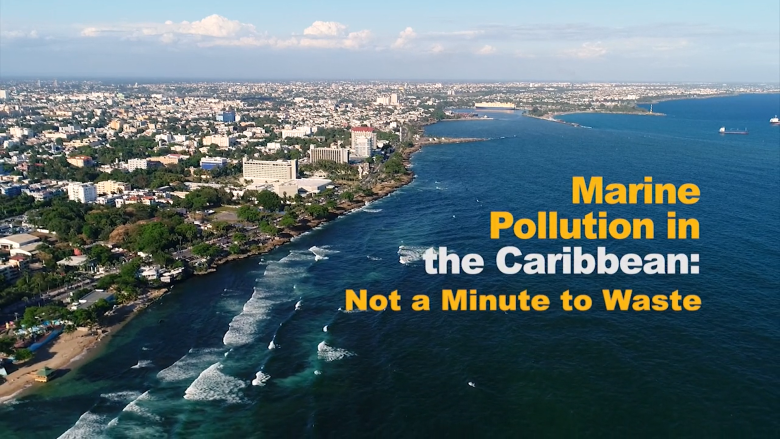The horizontally rectangular outdoor photograph captures an aerial view during the daytime using natural light. Dominated by a light blue sky filled with white clouds, the image shows the horizon seamlessly meeting deep blue waters. Along the upper right, a couple of boats are seen on the expansive blue sea. The lower left features waves crashing onto the beach, while the coastline is dotted with fluffy green treetops and numerous white buildings, indicating a heavily populated area. Yellow and white text, starting at the center right and moving downward, overlays the water, reading: "Marine pollution in the Caribbean: not a minute to waste." The stark contrast of the text against the rich blue water underscores the urgency of the message conveyed by the image.